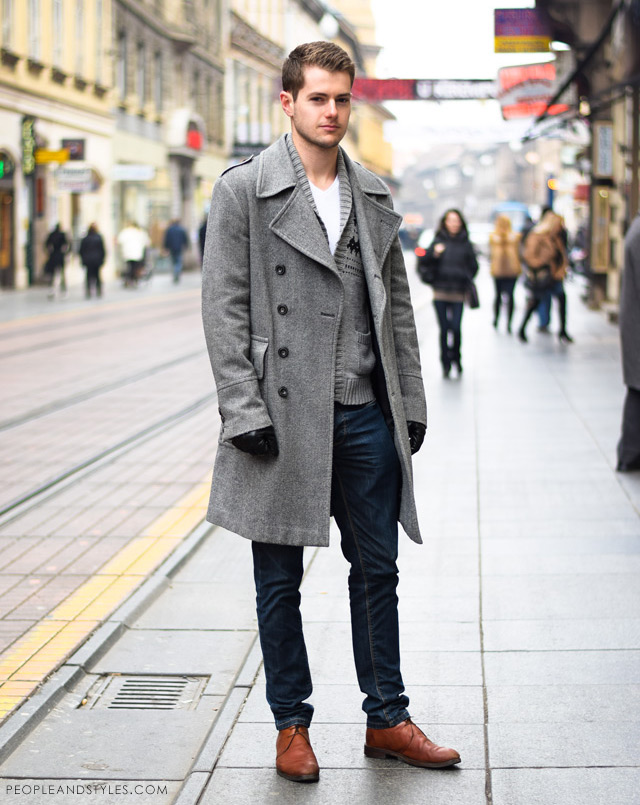The photograph captures a young white man, approximately in his early twenties, standing on a European-style pedestrian street that features tram tracks running through it. The man is prominently positioned off-center, slightly to the right, and is the focal point of the image, with the background elements artistically blurred to emphasize him. His attire includes light brown leather lace-up shoes, dark blue jeans, a white t-shirt, a grey vest, and a dark grey wool overcoat that reaches just above his knees. He also dons black leather gloves. His haircut is close on the sides with a slightly longer top. The street on which he stands has a grey sidewalk with a drainage grate near his right foot, and behind him, the brick road with tram tracks continues. Surrounding him are various multi-story buildings and signage, characteristically European, along with pedestrians walking, who are also blurred but identifiable, including a woman with long black hair dressed in black attire holding a red object. The man's neutral expression and direct gaze suggest he may be modeling his outfit, with the urban environment providing a dynamic backdrop.